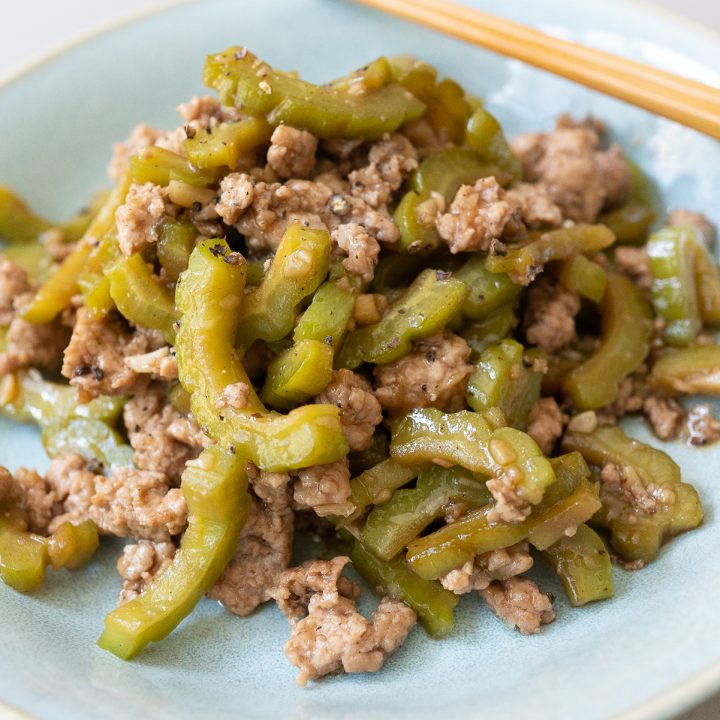This detailed image captures a close-up view of a plated dish, focusing primarily on the food itself while the background remains out of sight. The food is served on a light bluish plate, partially visible, with sections trimmed in a goldish-yellow hue, adding a subtle elegance to the presentation. The dish prominently features a green vegetable, likely sliced bell peppers, cut into semi-circular strips that stand out sharply against the plate, drawing immediate attention due to their vibrant color.

Mixed with the green vegetables is a lighter-colored cooked meat, possibly chicken, pork, or a type of ground meat. The meat appears seasoned with visible black and white specks dotting its surface, adding a textured visual interest. Scarce details indicate the presence of quinoa mixed into the dish, although this is less certain. There are no utensils in sight, emphasizing the food as the central focus of the photograph. The overall composition, with its mix of green vegetables and seasoned meat piled together, creates a visually appealing culinary presentation typical of professional food photography.